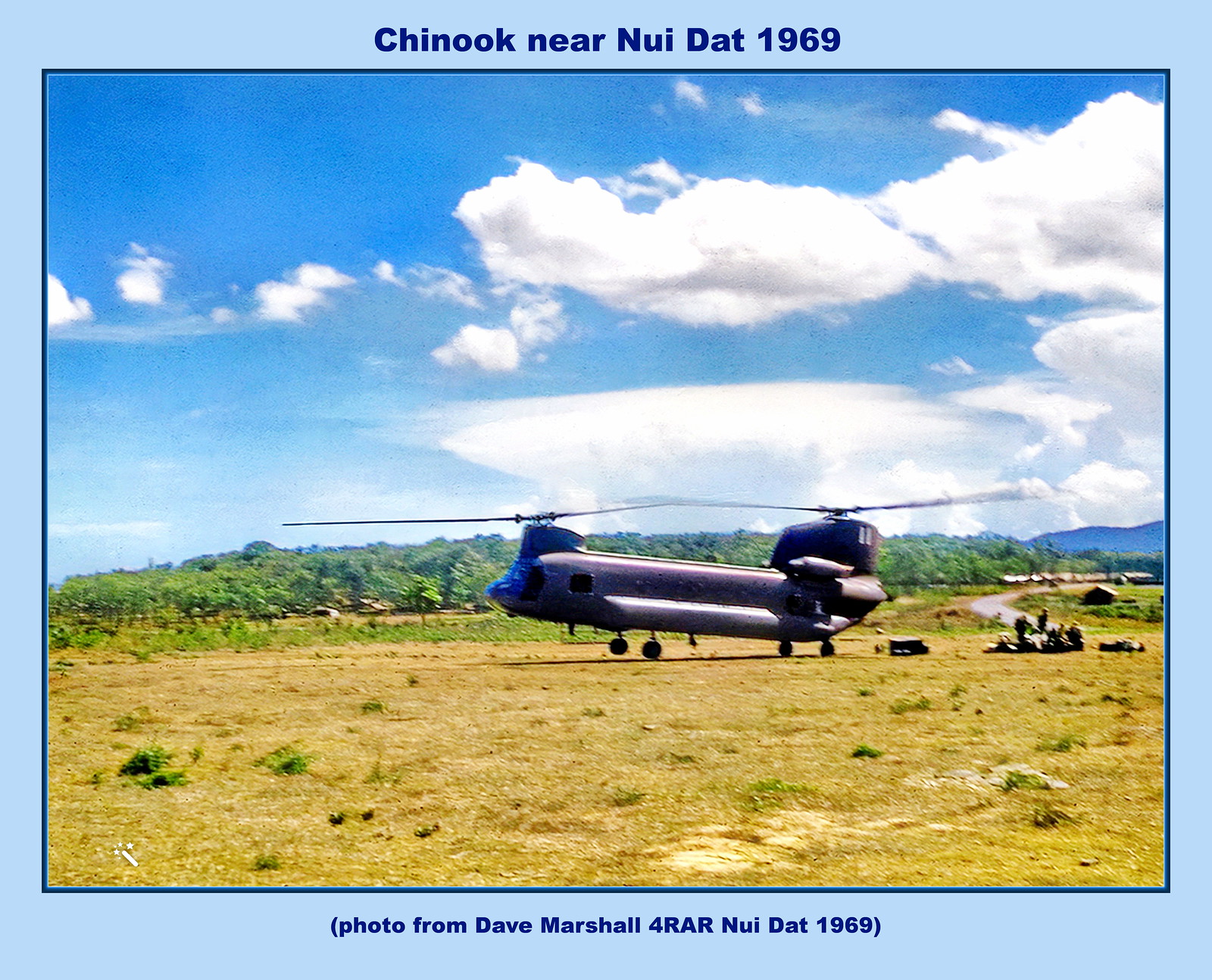The image depicts a military-style Chinook helicopter either taking off or landing in a grassy field near Nui Dat in 1969. The helicopter, with its front landing gear slightly off the ground, has its blades visibly in motion. The setting is a dirt field with patches of mostly dead grass and a dirt road behind the helicopter to its right. In the background, lush green trees and hills under a blue sky with large white clouds create a serene contrast to the scene. The photograph is framed within a wide vertical rectangle, with an additional black-bordered inner rectangle. At the top of the image, the text "Chinook near Nui Dat 1969" is prominently displayed, while at the bottom, it states, "Photo from Dave Marshall for RAR, Nui Dat 1969." The detailed context along with the surrounding elements underscores the historical and visual significance of this wartime snapshot.